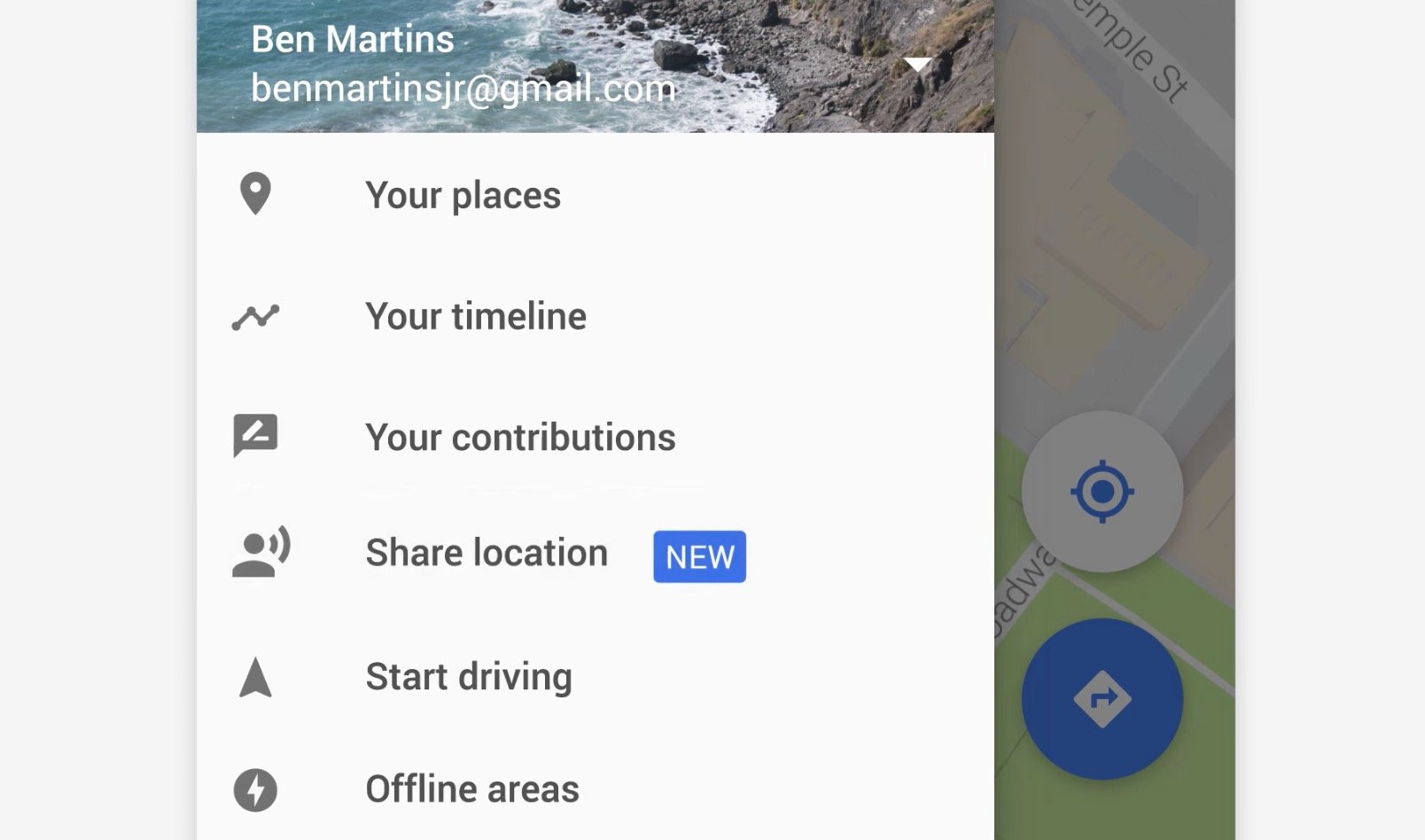The image is a screenshot bordered by light gray margins on both the left and right sides. At the top of the screenshot, there is a photograph of an ocean with waves crashing against a large set of high rocks, accompanied by smaller rocks below. Overlaid on this image, in white text, are the words "Ben Martens," with an email address beneath it that reads "benmartensjr," implying it could be "benmartensjr@gmail.com."

Below this, a white rectangular box displays the text "Your places," "Your timeline," and "Your contributions," with an adjacent option labeled "Share location" in blue. Next to this option is a blue square with the word "NEW" in capital white letters. The section below includes the options "Start driving" and "Offline areas."

On the right side of the screenshot, occupying the space from top to bottom, there is a map showing various streets. A gray circle with directional indicators (North, East, West, and South) sits prominently on the map. Beneath this, a blue circle contains a gray diamond, within which a blue arrow points to the right.